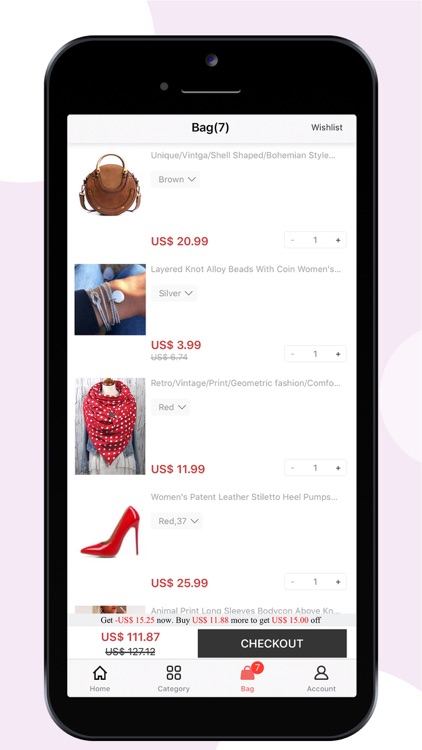The image depicts a phone screen displaying an online shopping cart. At the top of the screen, the header reads "Bag 7," and in the upper-right corner, it shows the "Wishlist" option. The cart contains a detailed list of items and their prices as follows:

1. **Unique Vintage Shell-Shaped Bohemian Style** (incomplete title): A brown item priced at $20.99.
2. **Layered Knot Alloy Beads with Coin Women's**: A silver item priced at $3.99.
3. **Retro Vintage Print Geometric Fashion Comfort** (incomplete title): A red scarf priced at $11.99.
4. **Women's Patent Leather Stiletto Heel Pumps**: A red pair of high-heeled shoes originally priced at $37.00, now $25.99.
5. **Animal Print Long Sleeves Bodycon Above** (incomplete title): A partially cut-off description with no visible price.

The total amount for the items in the shopping cart sums up to $111.87.